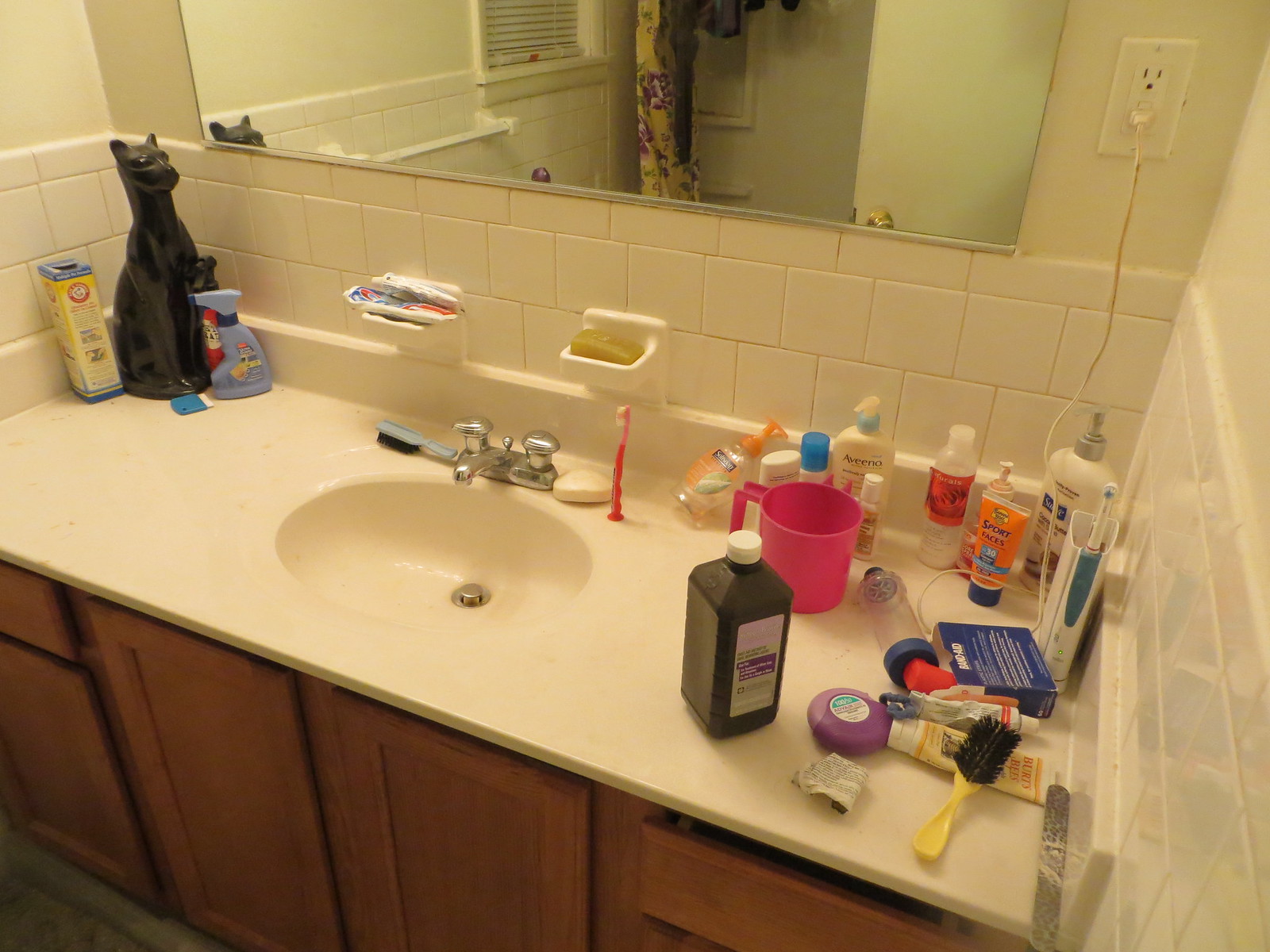This is a detailed photograph of a bathroom interior, likely taken at night given the absence of natural light from the window reflected in the mirror. The bathroom is illuminated by a bright fluorescent overhead light. The countertop features an oval basin with a modern mixer tap equipped with a push-down plug controlled by a small knob next to the taps. Above the white square-tiled backsplash, which extends approximately three tiles high from the countertop, the wall transitions to smooth, white paint. 

A prominent mirror without a frame covers a significant portion of the wall, reflecting a utility outlet with two sockets located in the upper right corner of the image, suitable for shavers or electric toothbrushes. The flooring is tiled in a dark gray hue, complementing the dark pine cabinetry below the counter, which comprises cupboards and two drawers.

The counter itself is cluttered with various items. In the top left corner stands a large black ceramic cat sculpture, surrounded by a few spray bottles and possibly a container of bath soap or bath salts. The space around the basin is occupied by a child's hairbrush to the left of the taps, and to the right, a slab of soap and a toothbrush with suction cups for easy attachment to the counter. Further back, a bottle of peroxide, additional children's brushes, a pink jug, some empty bottles, and various other bathroom products crowd the surface. Additionally, a toothbrush sits in a charging station in the back corner of the counter, indicating a well-used, functional family bathroom space.